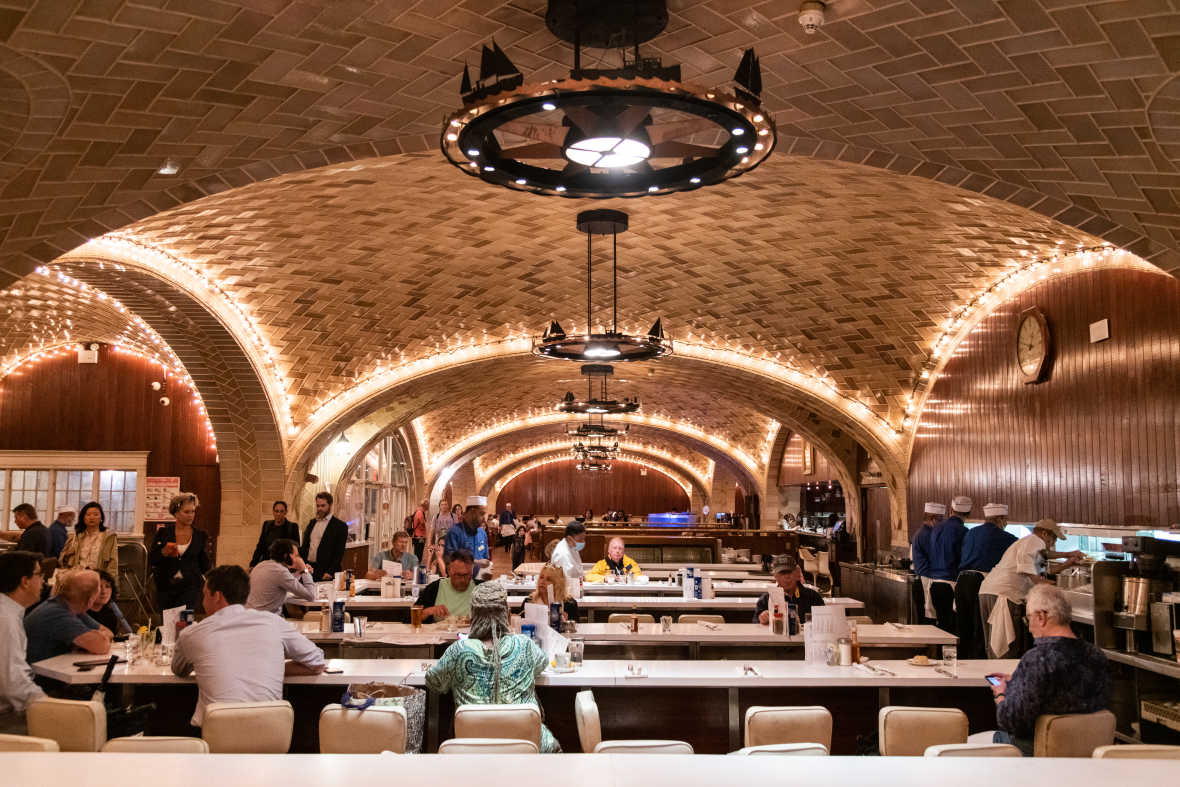The image depicts an elegant dining hall, possibly a part of a casino or a high-end restaurant, characterized by its unique dome-shaped ceiling with ambient lighting. The room is bustling with well-dressed patrons, suggesting an event or conference might be ongoing, hinting at a hotel setting. The walls are adorned with brown wood paneling, and a distinctive clock is situated on the right wall near several cooks in white hats. Long tables with white and brown tablecloths are spread across the room, each surrounded by brown chairs. Various people are seated or moving about, including a woman in green, a man in yellow facing the camera, a man in a dark blue shirt on his phone to the right, and a man in a whitish-gray shirt to the left. Additionally, some guests are seen walking to their tables, such as a woman in black and a suited man accompanied by another woman in black. Industrial chandeliers hang from the ceiling, illuminating the space, while a central pillar supports the dome architecture, dividing the room into distinct seating areas.